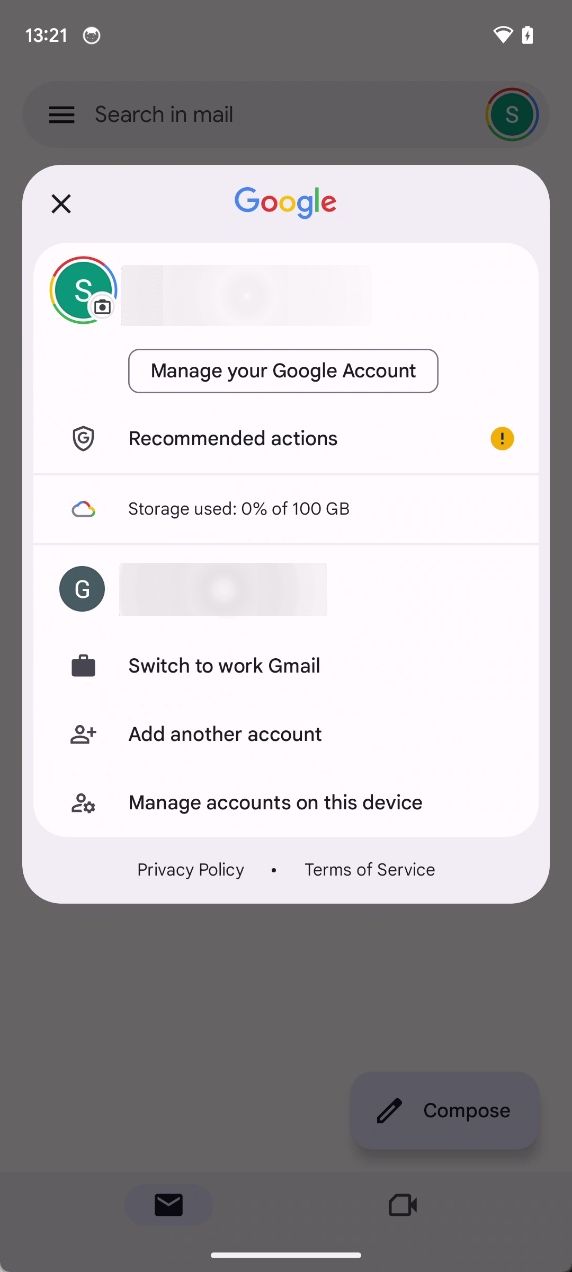This image is a screenshot of a Google services pop-up overlay on a mobile device. The background displays the Google search bar at the top, a clock showing 13:21, an almost full Wi-Fi signal icon, and a fully charged battery indicator. The overlay itself is rectangular with rounded corners, featuring the Google logo at the top center and an "S" within a circle surrounded by Google's four colors. Below the logo is an outlined rectangle indicating the manager's Google account.

Immediately following is a "G" inscribed inside a shield, next to which are "Recommended actions" with a black exclamation mark inside a yellow circle. Beneath this section is a cloud icon displaying "Storage used: 0% of 100 gigabytes." Below the storage information is a "G" inside a circle and an entirely blurred out field.

Further down, you'll find a briefcase icon with the text "Switch to work Gmail," a person icon with a plus sign labeled "Add another account," and a person icon combined with a gear indicating "Manage accounts on this device." At the bottom of the overlay are two link options: "Privacy Policy" and "Terms of Service," separated by a dot. The general background shows a blurred input field with the word "Compose" and a graded translucent covering.